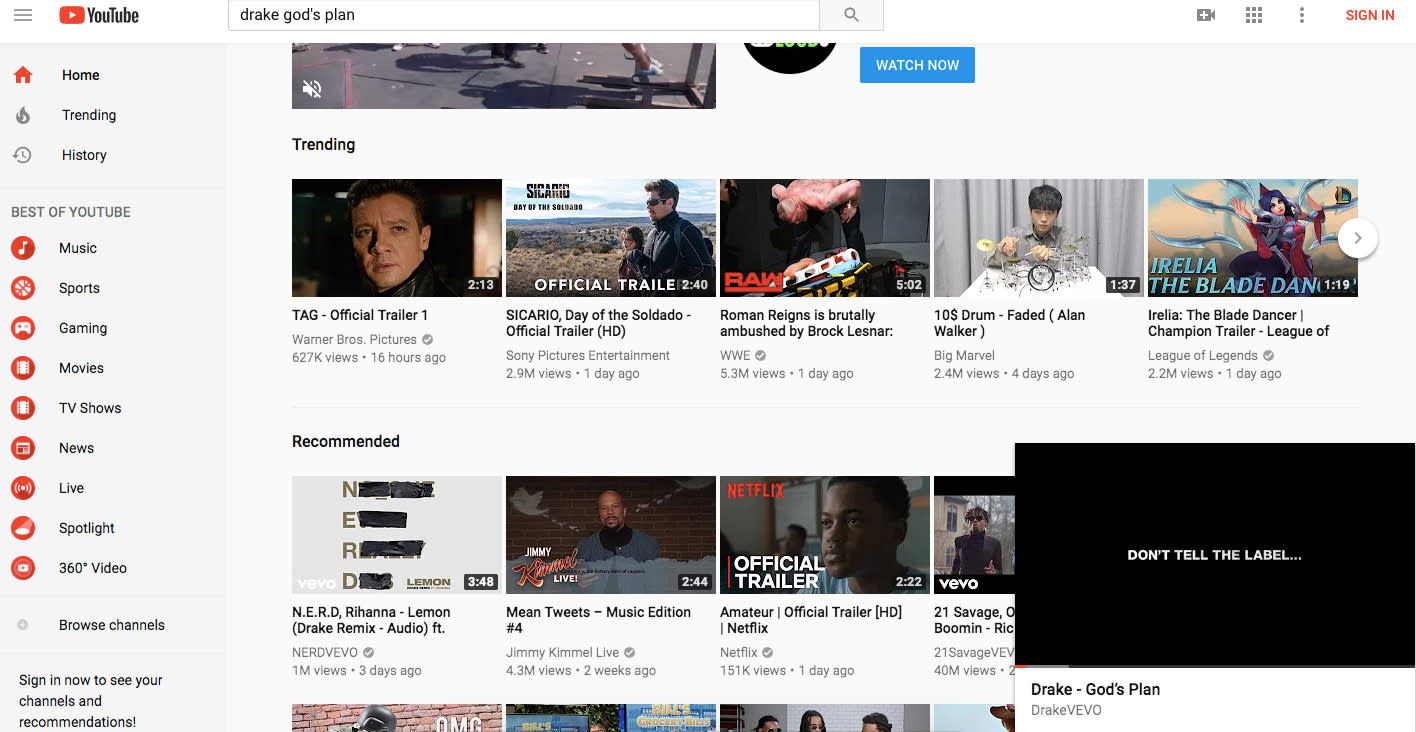The image depicts the YouTube platform interface. In the top left-hand corner, three black horizontal lines indicate a drop-down menu. To the right of this, the classic red, rounded rectangle with a white play button signifies the YouTube icon. Beside it, "YouTube" is written in their typical black logo, resembling the Impact font. Moving further right, there is a search bar with "Drake God's Plan" typed in, flanked by a light gray square icon featuring a medium gray magnifying glass symbolizing the search function. Further right, a dark gray camera icon with a white plus sign within it represents video upload. Adjacent to this, nine dots forming a gray square suggest another menu. Next to these, three vertical dots hint at an additional drop-down menu. Finally, on the far right, "SIGN IN" is written in small, capitalized red letters.

Below this section, a strip features five video thumbnails. The first thumbnail displays bold black text reading "TAG - Official Trailer 1." Next to this, an image of a man and possibly a shorter man or boy against a landscape background with "Official Trailer" written in white. Below this, the title "Sicario: Day of the Soldado - Official Trailer (HD)" is in bold black lettering. To the right, an image possibly of an instrument or toy with a pink cloud at the top, and in the bottom left corner, bold blocky red text reads "RAW." The accompanying title, "Roman Reigns is Brutally Ambushed by Brock Lesnar," is visible below.